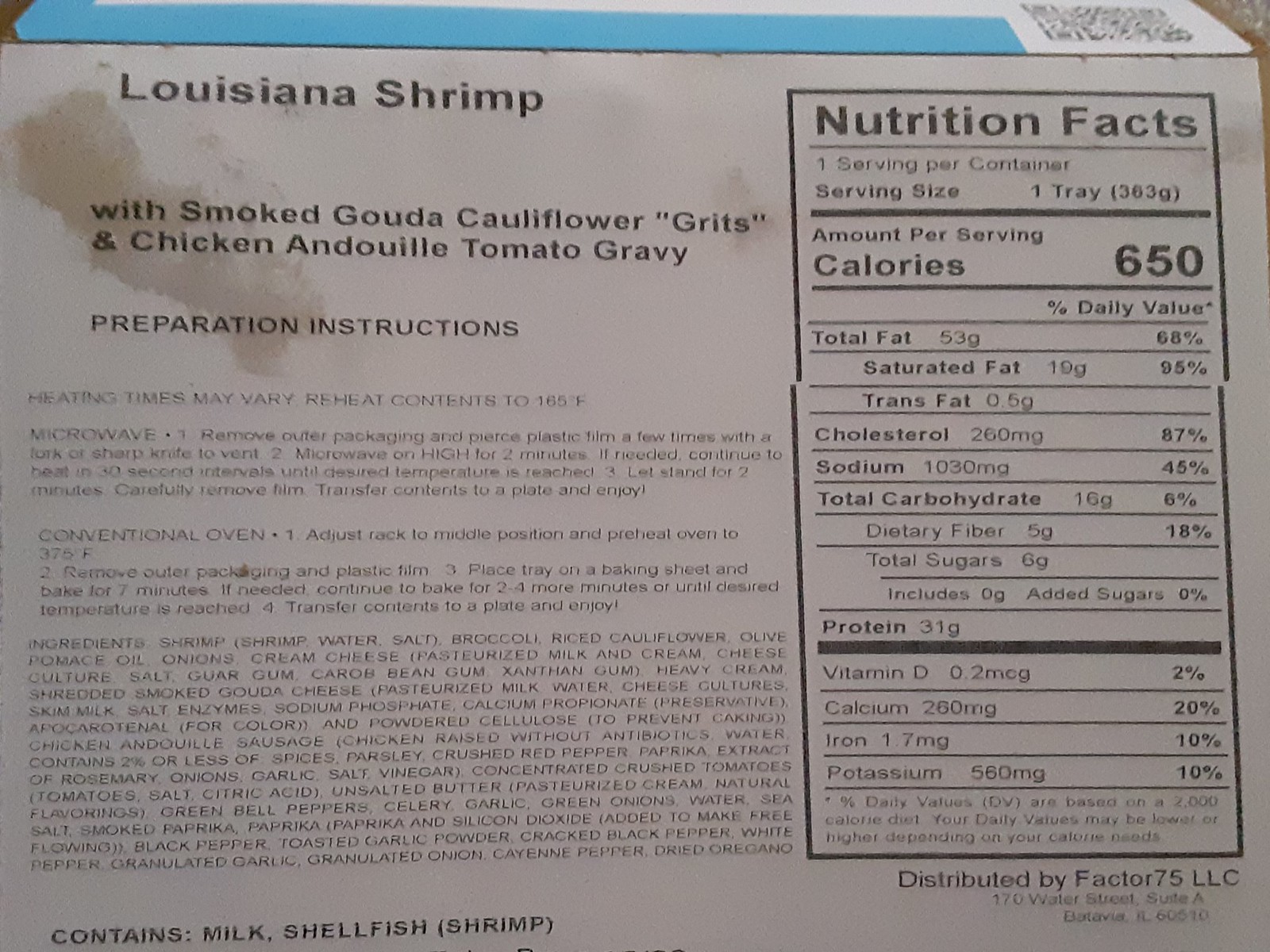This is a detailed photograph depicting the nutritional information and ingredients label for Louisiana Shrimp with Smoked Gouda, Cauliflower Grits, and Chicken Andouille Tomato Gravy. The packaging has a gray color scheme with a blue stripe, and includes a noticeable QR code in the upper right corner. A host of ingredients fills a third of the left side of the image.

The meal, which exudes a distinctly Cajun and Southern flair, is described as flavorful and spicy. Heating instructions recommend reheating the contents to 165 degrees Fahrenheit for safe consumption, with specifics for both conventional oven and microwave options.

Nutritionally, the meal contains 650 calories per serving, with the serving size noted as one tray, and there is only one serving per container. The packaging also highlights potential allergens, including milk and shellfish (specifically shrimp). Additionally, there is an emphasis on the necessity of safe reheating practices, indicating that heating times may vary.

This product is distributed by Factor 75 LLC, located at 170 Water Street, Suite A, in what appears to be Batavia, Florida, ZIP code 60510, although the city name is not entirely clear.

In summary, the packaging provides a complete and appetizing overview of a high-calorie, distinctly Cajun shrimp dish with diverse flavor elements and clear instructions for safe preparation.